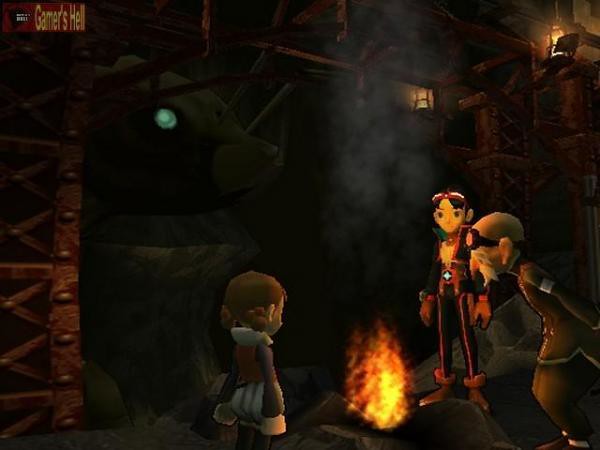In this screenshot from a polygonal-style video game, reminiscent of an early 2000s aesthetic, three animated characters are gathered around a small campfire, within a dimly lit, industrial-like setting. The scene includes rusty metal frames, structures, and pipes, suggesting an old factory or basement environment. The background also features hanging lanterns and a circle of light to the left, setting a nighttime ambiance.

On the left side of the campfire stands a short girl, identifiable by her distinct hairstyle with hair tied into little buns at the back of her head. She is dressed in a long-sleeve puffy outfit with a stand-up collar, featuring purple sleeves with woolly cuffs and vertical stripes along her coat. To the right of the campfire, there's an older, bald man with a white beard, glasses perched on his forehead, a pointy nose, and chin. He is hunched over with his hands behind his back, wearing brown overalls with a white stripe around his upper left arm, and appears to be gazing into the fire. Opposite the old man stands a tall, skinny woman who looks to be wearing athletic gear, possibly a martial arts uniform, with a headband and a notable blue light on her stomach. The trio is illuminated primarily by the fire's glow against the dark surroundings. A caption at the top left corner of the screen reads "Gamer's Hell."